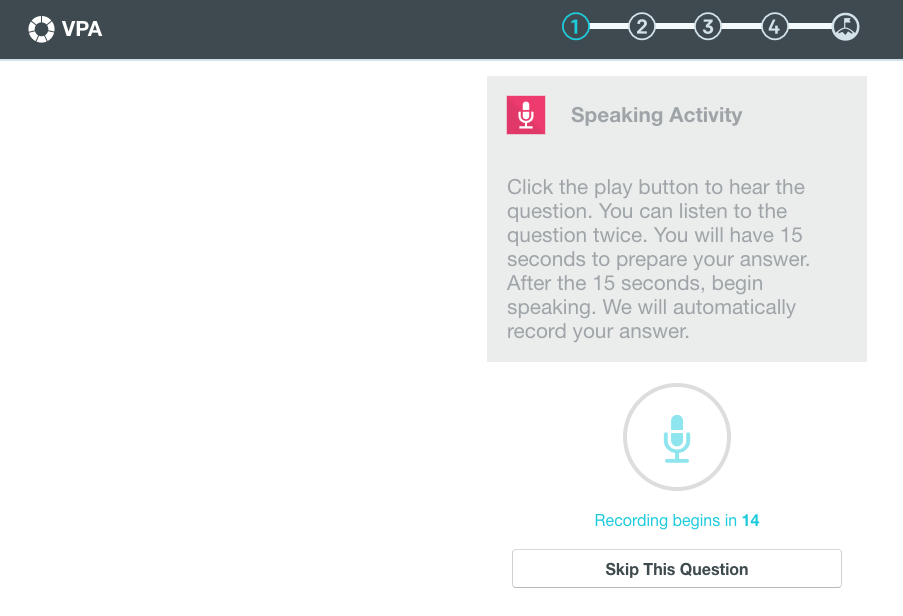The image showcases a digital cockpit interface prominently labeled "VPA" in the top left corner. The interface features a multitude of numbered elements: seven distinct icons numbered from 1 to 7, a wheel, and a prominent blue circle also marked with the number 1. Additionally, it includes a self-printing flag symbol and a section in the background with a wiring schematic. 

On the top left, there is a detailed gray square housing a red square that contains a microphone icon. The entire interface is predominantly gray, enhancing visibility for various textual instructions present within the display.

Text on the screen guides the user through an interview process: "Click the play button to hear the question. You can listen to the question twice. You will have 15 seconds to prepare your answer, after which we will automatically record your response." This setup suggests that the interface might be used for an automated interview scenario where questions are played back, and responses are recorded.

In the center of the interface is a gray circle with blue highlighting, featuring a blue microphone icon and blue text that reads "Recording because of routine." At the bottom right, there is a final element: a button labeled "Skip this question."